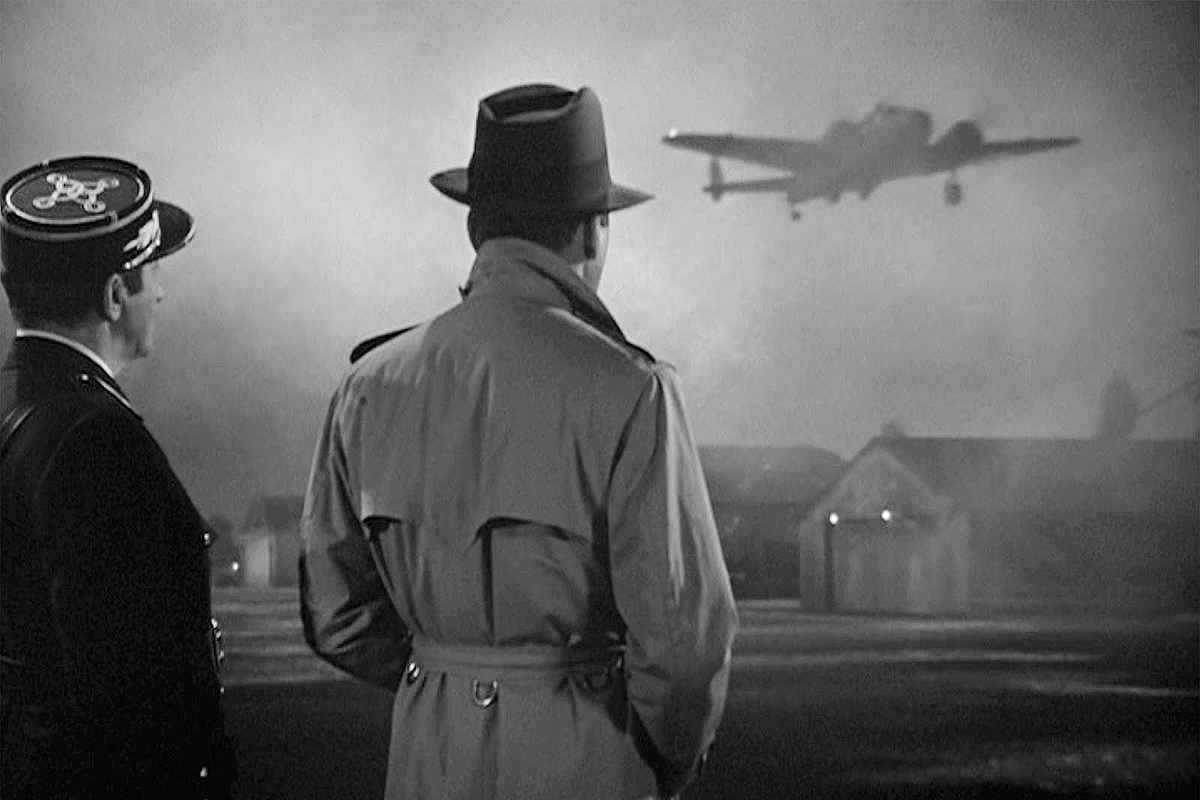This black and white still from the final scene of the movie *Casablanca* captures the poignant farewell at the foggy airport. Humphrey Bogart, portraying Rick, stands with his hands in his pockets, clad in a gray trench coat with the collar turned up and his signature fedora. Beside him is Louis, the French policeman, dressed in a World War II-era uniform. Both characters are viewed from behind as they watch the Laszlos' plane take off into the night. The scene is set against a backdrop of cloudy, smoky skies, with indistinct airport buildings visible in the distance, encapsulating the somber mood and atmospheric conditions pivotal to this iconic cinematic moment.